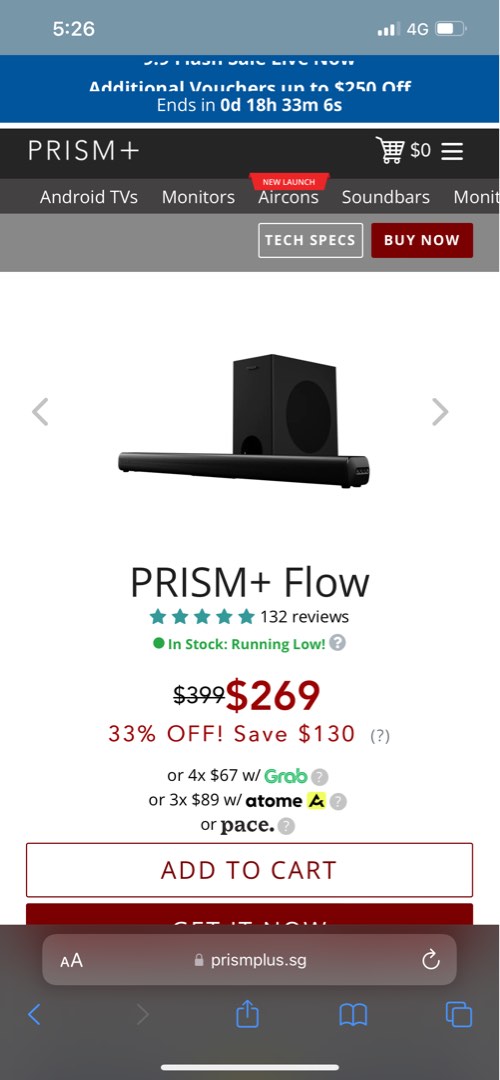The image is a screenshot from a cell phone displaying an online shopping page. At the top of the screen, there's a banner announcing "Additional Vouchers up to $250 Off" with a countdown timer showing "Ends in 0 days, 18 hours, 33 minutes, and 6 seconds". Below the banner, the user is viewing a product called "Prism+ Flow". The product has amassed 132 reviews and boasts a perfect 5-star rating. It is listed as in stock but noted to be running low. Originally priced at $399, the product is on sale for $269, with this price highlighted in red. Additionally, there is a red tag indicating "33% Off!" and a note mentioning that you save $130. Below the price, there are payment options: "4 payments of $67 with Grab" or "3 payments of $89 with Atome or Pace". At the bottom of the screen, there's a prominent white button with red text reading "Add to Cart". The website URL "prismplus.sg" is displayed at the very bottom of the image.